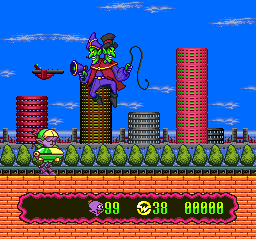Screenshot of a mobile game featuring an intricate landscape and various elements: At the bottom of the image, there are orange blocks followed by a pink scoreboard displaying "99" next to a peculiar purple character. Nearby, a circle with a "W" signifies a score of 38. Below the scoreboard, a sequence of five zeros is displayed in green text. Above these numerical elements, there's a patch of green bushes and a secondary character navigating alongside them. The background showcases a cityscape with four distinct buildings: an all-red structure, a smaller gray building, a black-and-green edifice, and a larger pinkish-purple construction. Prominently featured are two two-headed characters resembling the Joker, one wielding a whip and the other a horn. The sky overhead is a deep blue, dotted with white clouds, completing the atmospheric scene of this enigmatic mobile game.